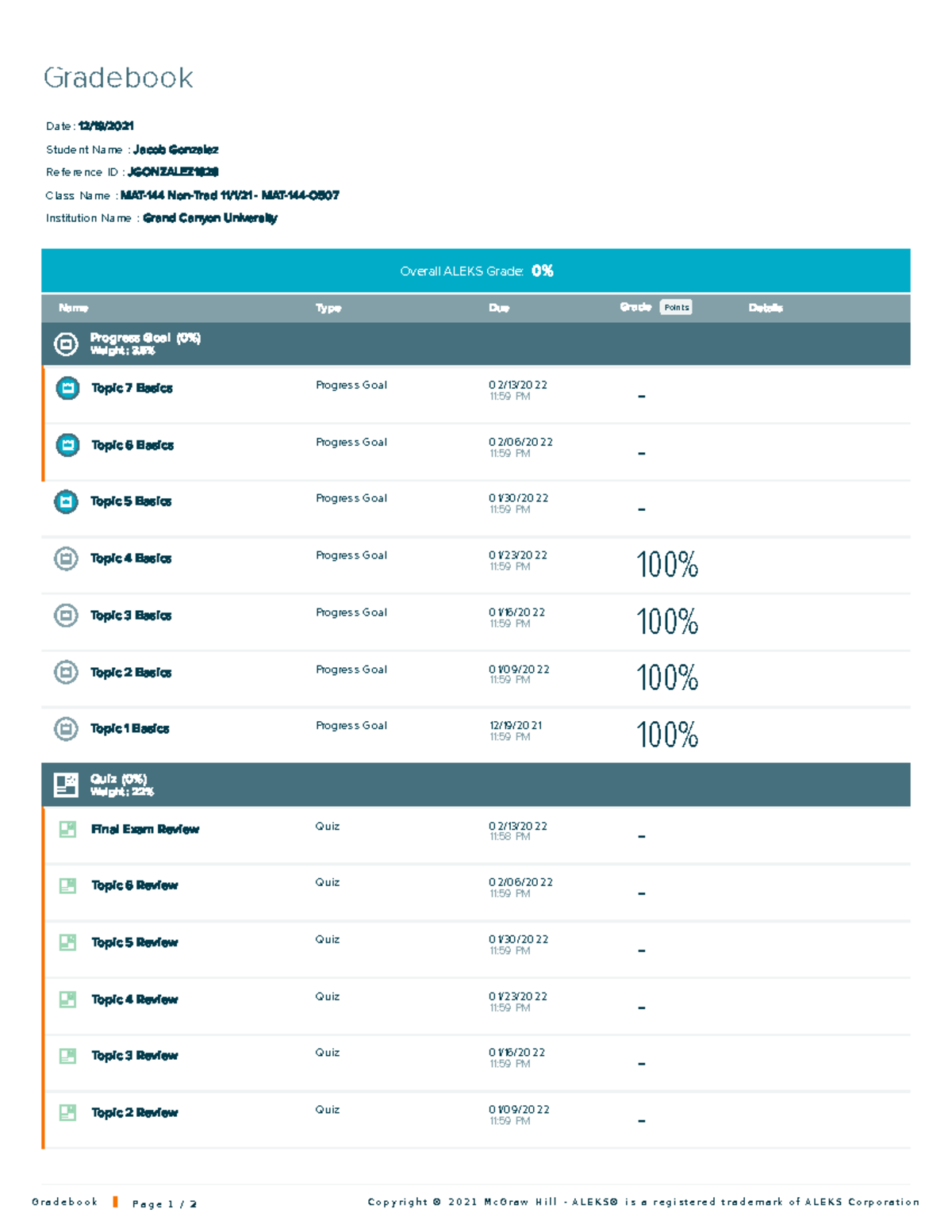This image is a screenshot of a digital gradebook interface, displayed within a vertically elongated rectangular frame set against a white background. At the top left corner, the gray header reads "Gradebook." Below this header, the text "Date: 12-19-2021" is displayed.

The student's name, "Jacob Gonzales," is prominently highlighted in bold dark teal text. His reference ID, "JGonzales1828," is listed next to it. The class information includes the class name "Matt144" with the designation "Non-Trad," followed by the class date "11-1-21." The institution is identified as "Grand Canyon University."

Beneath this information is a teal-colored banner stating, "Overall Alex Grade: 0%." Following this, there is a gray banner with white text headings that read from left to right: "Name," "Type," "Due," "Grade," "Points," and "Details." Below this banner lies a dark green box with white text, indicating "Progress Goal: 0%" and "Weight: 3.5%."